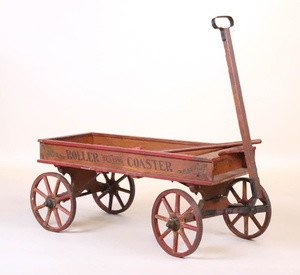In this rectangular image set against a stark white floor and background, a vintage, rusted children's wagon is displayed prominently. This classic red wagon, appearing well over a century old, features four spoked wheels and exhibits extensive rust, particularly on its underside carriage. The rectangular body of the wagon maintains its red color but shows patches of rust, most notably in the corners. On the east-facing side, faded capital letters spell out "ROLLER COASTER." A red handle, positioned upright on the right side, includes an open grip area, inviting one to imagine the days when this piece of history was a beloved toy.